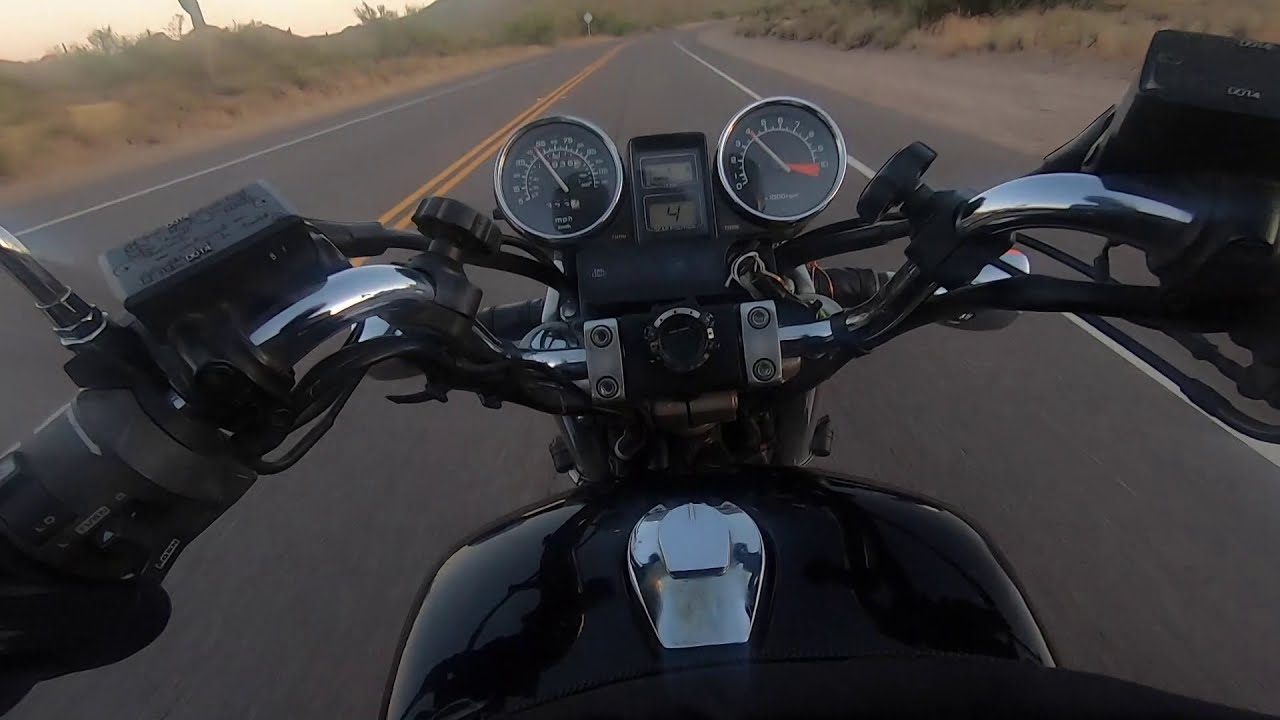The photograph captures the view from the driver’s perspective on a black motorcycle traveling down a paved two-lane road. The scene reveals a somewhat deserted, likely western state landscape with dry scrub brush lining the road and an overcast sky. The focus is on the motorcycle’s handlebars and controls. The dashboard shows two dials; the left one indicates speed, showing around 50 miles per hour, while the right one shows RPM, reading close to 4,000. Glimpses of the driver's gloved hands are visible—the left in the bottom left corner and the right near the top right. The polished metal parts of the motorcycle reflect light, adding shine to the black and chrome details. The center features a silver gas cap and a digital readout with a '4', though its significance is unclear. The road features a double yellow line, indicating a no-passing zone, contributing to the overall feeling of solitude and openness.